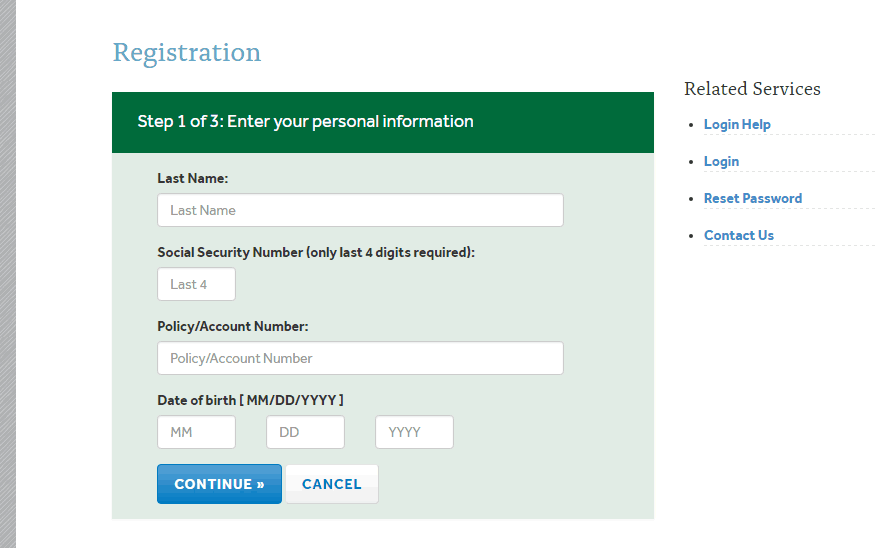The image displays a registration form interface. Starting in the upper left corner, the word "Registration" is highlighted in blue text. To the far left, there is a long, vertical, thin, gray rectangle. Below the "Registration" title, a green rectangle labeled "Step 1 of 3" is displayed. This step instructs the user to "Enter your personal information," indicated by two small dots vertically aligned.

Under this instruction, in a lighter green font, it says "Last Name," accompanied by a long rectangular input field that also says "Last Name" as placeholder text. Following this, the user is prompted to enter their "Social Security Number," with a note in parentheses indicating that "only the last four digits are required." Another rectangular input field labeled "Last Four" is provided here.

Next, the form prompts for the "Policy/Account Number," again indicated by two small vertically aligned dots. This field is represented by a large white rectangle labeled "Policy/Account Number." Below this, in black text, the form asks for the "Date of Birth" with the format specified in parentheses as "MM-DD-YYYY." Three small squares are provided underneath to enter the month, day, and year respectively.

At the bottom of the form, there are two buttons for the user to interact: a "Continue" button inside a blue box and a "Cancel" button inside a white box. Over on the right side of the form, there is a section titled "Related Services," listing the following items sequentially: "Login Help," "Login," "Reset Password," and "Contact Us."